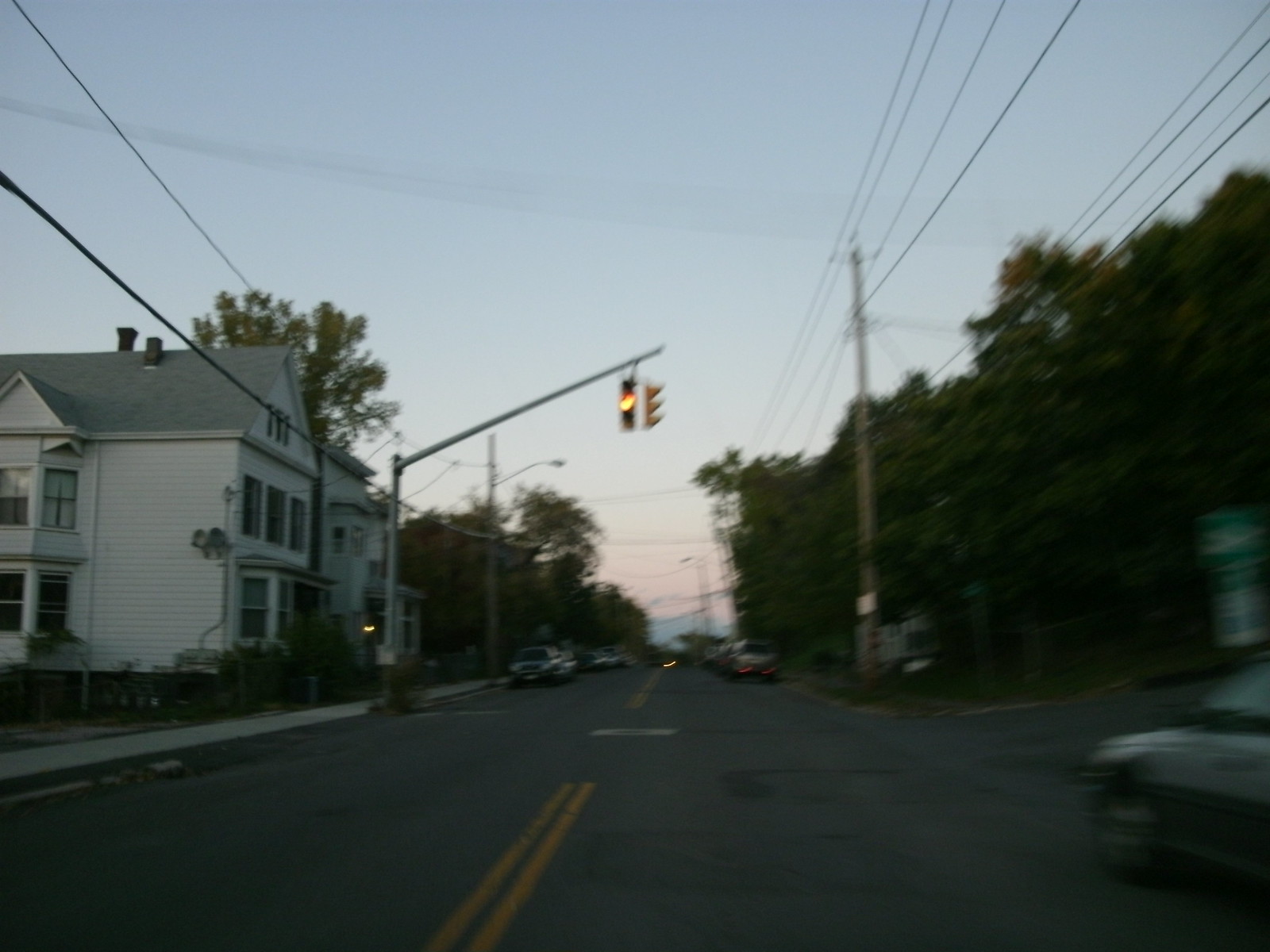A blurred photograph captures a quiet street scene at dusk, taken from inside a moving car. The sun is setting, casting a soft, dim light over the neighborhood. The car has slowed down or is briefly stopped, allowing a streetlight overhead to cast a warm yellow glow onto the road. Another car approaches from the right, where a side street veers off, leading deeper into a wooded area dense with trees.

Up ahead, cars are parked on both sides of the road, contributing to the lived-in feel of the area. To the left, two houses with white siding stand prominently. These homes, each boasting at least two and a half to three stories including attic spaces, feature older architectural details like protruding windows, hinting at a construction period from the early to mid-1900s. A sidewalk runs alongside these homes, adding a quaint, pedestrian-friendly charm to this seemingly historic neighborhood. The scene evokes a sense of nostalgia and calm, framed by the twilight hour.